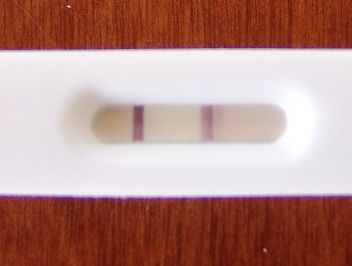The photograph is in a horizontal (landscape) orientation, captured on a reddish-brown wood-grained table. At the center of the image lies a rectangular white plate that spans the entire width of the photo. Positioned prominently on the plate is a long, capsule-shaped object, which resembles a sausage. The object has rounded edges and features a gradient of colors. Starting from one end, it displays a light cream color, followed by a red ring. The central portion of the object is white, encircled by another ring in a lighter, brick-like shade. The remaining part transitions to a cream or beige hue, creating a visually striking contrast against the white plate and wooden table.